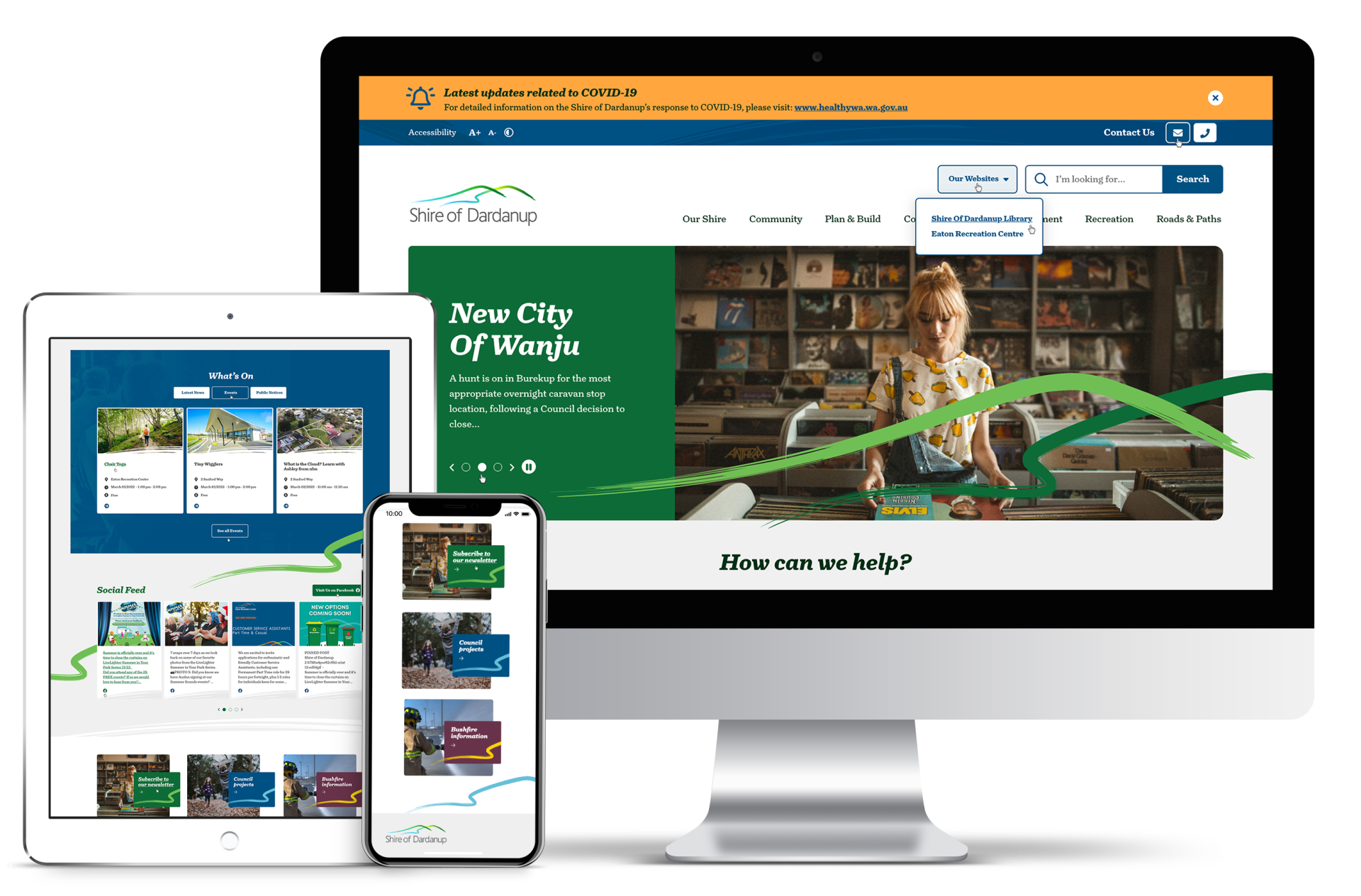This image showcases the completed website design for the "Shire of Dardenup" and the "New City of Wanju." It appears to be a mockup presenting how the website would look across different devices. The central focus is a desktop computer, which looks like an iMac, demonstrating the detailed website interface. To the left of the iMac, there's an iPad displaying the tablet version of the site, and further left, a smartphone showcases the mobile layout. Each of these devices has their screens digitally altered, likely via Photoshop, to illustrate the website's responsive design. The desktop version reveals the most intricate details, while the tablet retains some of this detail, and the mobile version simplifies the content significantly, with most elements rearranged into a portrait mode. It appears there is also an image suggesting a bookstore, indicating that part of the website's functionality may relate to a bookstore or a similar entity.